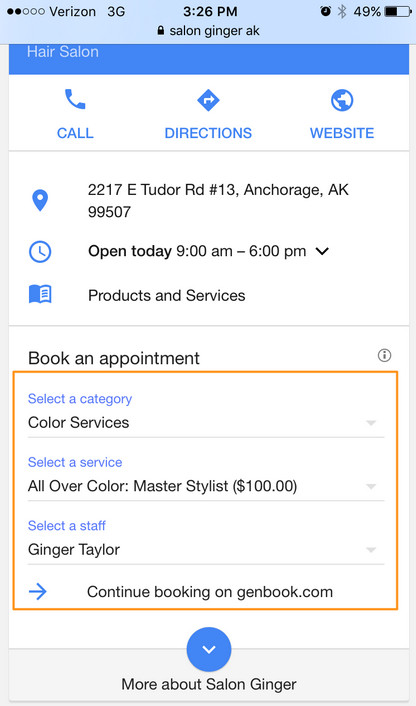This screenshot captures a Google search page for the business "Salon Ginger AK." The phone's banner at the top of the screenshot is light blue. On the top left, the signal strength is indicated by two out of five circles, next to the carrier name "Verizon" in black and "3G" in black. The center of the banner shows the time as "3:26 PM" in bold. On the right side, it displays the device information, including a battery percentage of 49%, along with icons for Bluetooth and an alarm, both of which are enabled. Additionally, at the bottom center of the banner, there is a lock icon accompanied by the text "Salon Ginger AK."

Below the banner, the search page information is on a white background. At the top, there is a blue header labeled "Hair Salon." The view is scrolled down, showing that the image of the hair salon is missing. There are three prominent options in a large white box: "Call," "Directions," and "Website."

Further down, three lines of information with corresponding icons on the left provide essential details. The first line has a location icon followed by the address, the second shows a clock icon with the business hours, and the third features a magazine icon with the text "Products and Services."

Underneath this, another large white box titled "Book an Appointment" appears on the top left in black text. Below this are three dropdown boxes in blue for booking services, labeled "Select a Category," with "Color Services" selected, "Select a Service," with "All Over Color" selected, and "Select a Staff," where one of the staff member's names is chosen. Finally, at the bottom of this section, it instructs users to "Continue Booking on Genbook.com."